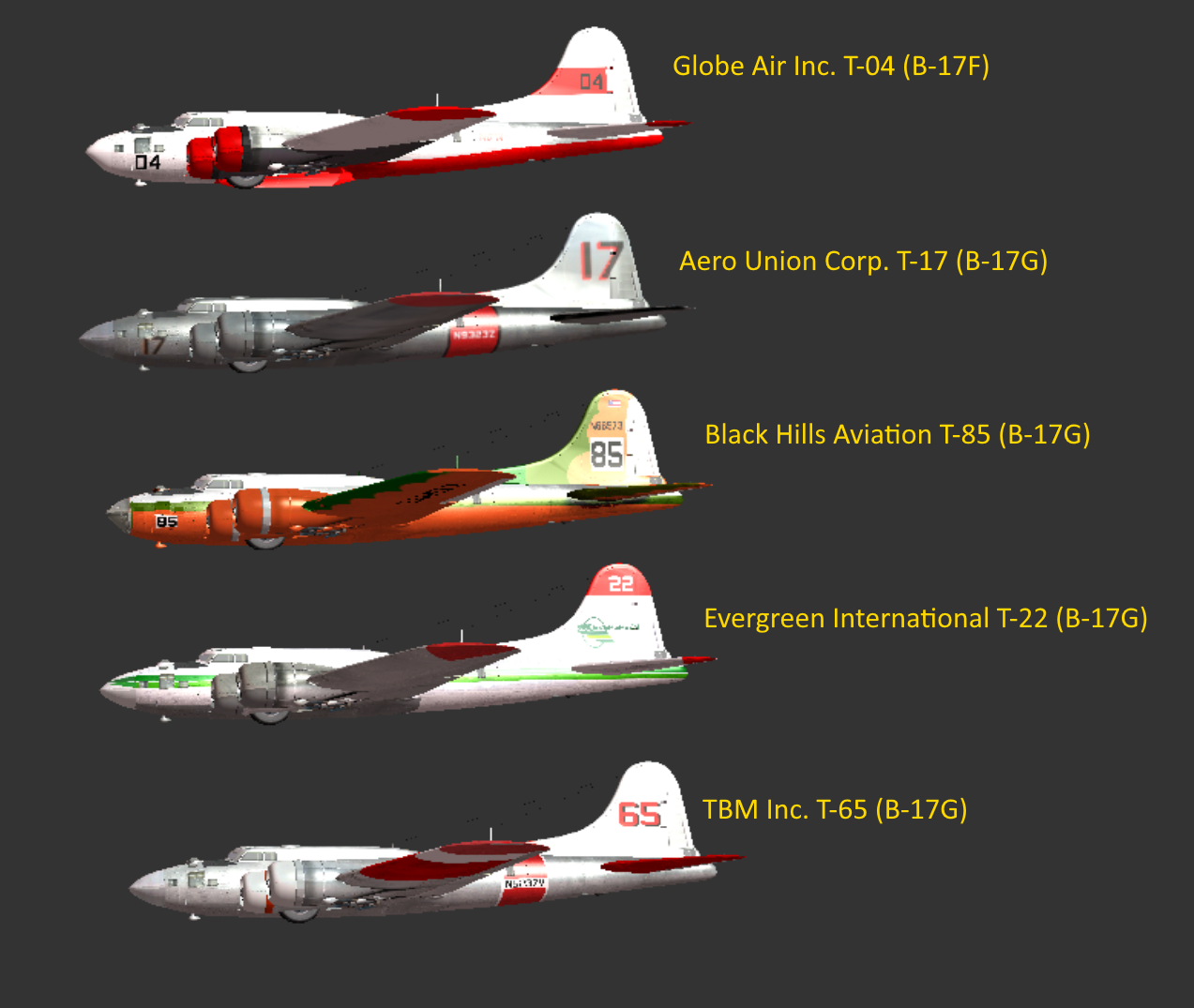The image is a detailed 3D illustration showcasing the evolution of airplane liveries against a solid dark gray background. It features five airplanes, each representative of a different model and era, yet all sharing a similar basic design, reminiscent of large aircraft with rounded tails, two engines per wing, and a gently pointed nose.

At the top, the first plane is notably characterized by red accents on its fuselage and lower body, annotated with "Globe Air Inc. T-04B17F" in yellow text. Below it, the second plane is primarily a silvery gray with red wingtips and trim, bearing the identifier "Aero Union Corporation T-17B17G" in yellow, with a large "17" visible on its tail. 

The third plane exudes an orangey-red hue, marked with "85" on its tail and labeled "Black Hills Aviation T-85B17G" in yellow lettering. Further down, the fourth aircraft is predominantly white, featuring a distinctive green stripe down the middle and a "22" on its tail; it is identified as "Evergreen International T-22B17G". 

Lastly, the bottom plane is mostly white with red accents, particularly on the wings, and has "65" on its tail, with the caption "TBM Inc. T-65B17G" in yellow.

Together, these elements offer a rich, informative glimpse into the variety and history of plane liveries across different aviation companies and models.